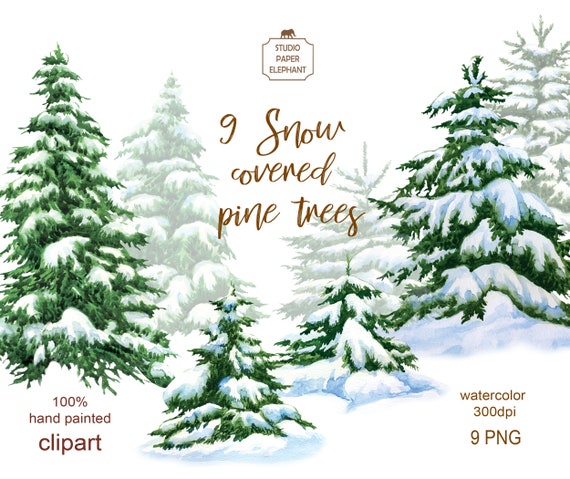The image is an idyllic, hand-painted clip art design by Studio Paper Elephant, prominently featuring their logo at the top center with a small elephant figure and a patterned frame. The text "Studio Paper Elephant" is written in a strange, cartoonish font followed by "Nine Snow-Covered Pine Trees" in a stylistic, cursive style. The scene showcases a collection of nine green, snow-draped pine trees, including four detailed, darker ones in the foreground and three lighter, more muted trees in the background, set against a misty, daytime backdrop. Additionally, there are two smaller pine trees adding variety to the composition. The bottom left corner of the image reads "100% Hand Painted Clip Art" while the bottom right corner specifies "Watercolor, 300 DPI, 9 PNG." This serene and picturesque artwork evokes a classic, wintry Christmas setting.